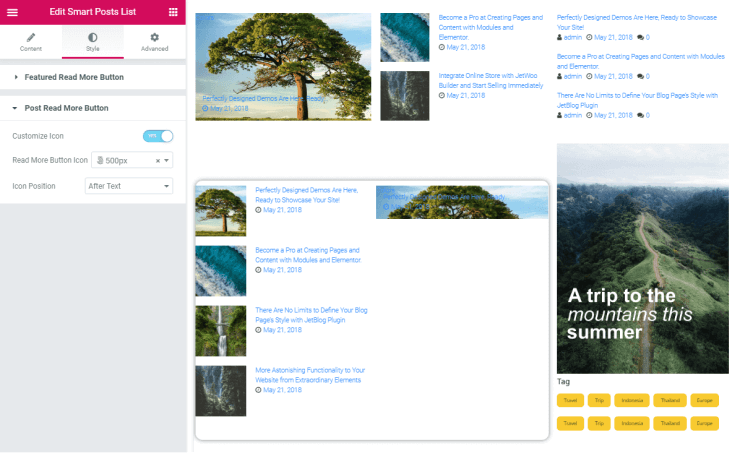This landscape-oriented image appears to showcase a search result related to vacation rentals, embedded within a photo and caption editing interface. 

In the top left section of the interface, a pink horizontal border frames a handwritten menu in white, accompanied by the text "Edit Smart Post List." Adjacent to this, a grid view option is also visible. 

Beneath this section, a white bar provides various options labeled "Content," "Style," and "Advanced." Moving further down, there's a customizable "Featured Read More Button" and a "Post Read More Button." This section includes toggles and settings for customization, with the toggle switch currently set to "Yes." 

To the right, a prominent image of a tree with green leaves and a sturdy trunk is displayed. Additional smaller pictures featuring trees and bodies of water are accompanied by blue text.

Directly beneath, another image of the same tree is shown, with a caption dated May 21st, 2018. This part of the interface includes similar photos, each with varying captions that appear to have been edited.

To the right again, a striking image depicts the top of a mountain with a pathway flanked by trees. This section is overlaid with the text "A Trip to the Mountains This Summer," written in white, and includes various tags for categorization.

Overall, the image highlights a complex photo and caption editing system designed for a website, displaying multiple elements such as images, customizable buttons, captions, and editing options.